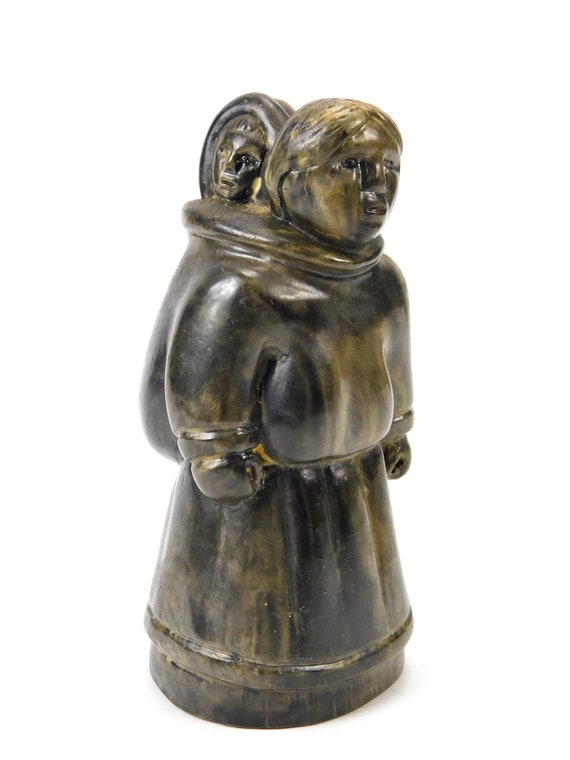The image depicts an intricately crafted figurine that appears to be carved from a material that resembles dark brass, bone, or perhaps a composite with a wood-like appearance, featuring shades of dark and lighter brown. The sculpture portrays a female figure dressed in traditional attire, a long gown with long sleeves that reach her wrists, and a belt cinched around her waist. This figure has flat hair and is facing toward the right side of the image. She carries a child on her back, who is bundled up with a hood over their head and secured with a scarf-like carrier attached to the mother. The surface of the figurine has a slight shine, indicating its aged yet well-preserved condition, and it stands on a plain white background which emphasizes its details.